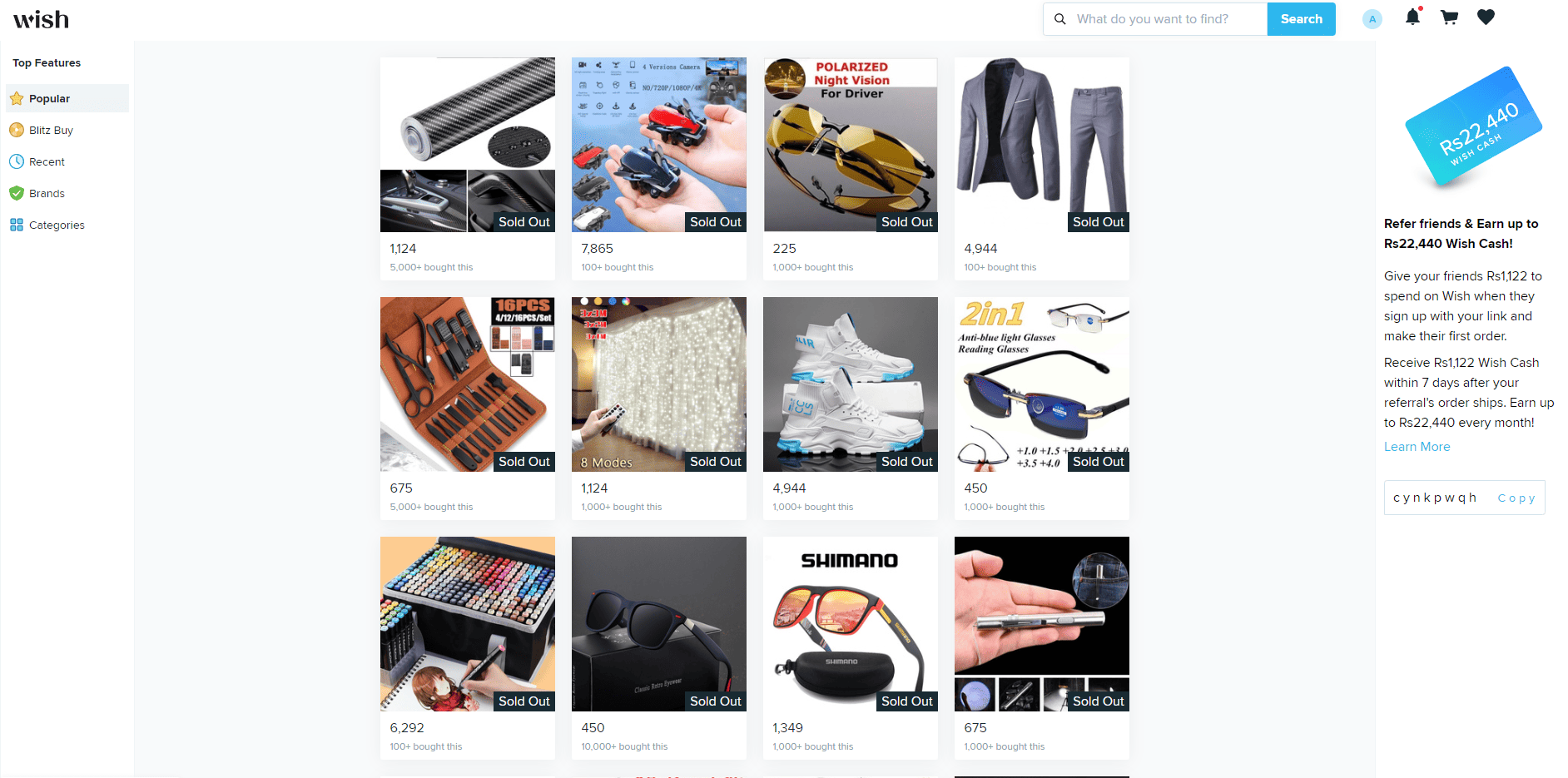A detailed screenshot with a gray background features the following elements, structured from left to right:

- On the top left corner, the Wish logo is prominently displayed.
- Adjacent to the right is a search bar with a magnifying glass icon and a blue rectangle containing the word "Search" in white text.
- Further right, a notification bell icon features a red dot indicating new notifications.
- Next to the notification bell, there is a shopping cart icon, followed by a heart icon which typically represents saved or liked items.
- Below these, there appears to be a credit card-like graphic with a promotional message reading, "Refer friends and earn up to RS-22440 Wish Cash," suggesting a referral reward program. A link with the text "Learn more" in blue offers additional information about this promotion.
- Toward the bottom of this section, a code presumably comprised of the letters CYN, KPW, QH, and spelled out in blue is displayed, which might be a referral or promotional code.

In the main section of the screenshot, there are 12 images of different items arranged in a grid format:

1. The first image seems to depict a car-related item.
2. The second image shows what appears to be a gadget, likely also car-related.
3. The third image displays a pair of sunglasses.
4. The fourth image features a gray suit.

Each of these images is overlaid with the text "Sold Out," indicating none of these items are currently available for purchase.